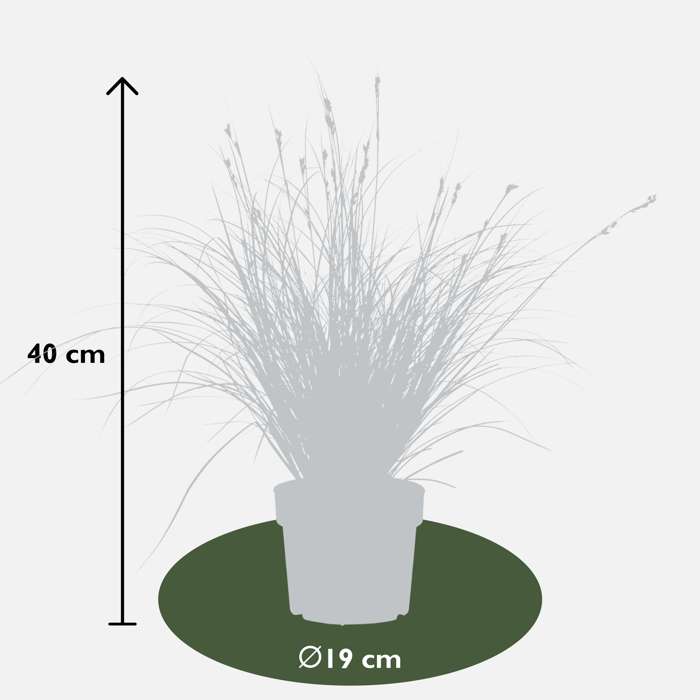This image appears to be a digitally rendered diagram, likely reminiscent of an illustration from a textbook, designed to measure plant height. The background is predominantly gray, featuring a central green circle or disc at the bottom. This green circle contains a white circle with a line through it, marked with the label "19 cm." Positioned to the left of the green circle, an arrow points upwards and is labeled with "40 cm" in black text. Rising from the green circle is a gray pot with a plant. The plant and pot are entirely gray, depicted in such a way that they appear as shadowy or silhouetted forms without any color. The plant itself looks whispery, almost like grass with little springs or budding flowers, but with no detailed coloration. The minimalistic color palette of the image includes only green for the disc, white for the 19 cm label, and black for the 40 cm label and arrow, highlighting the measurement aspects of the illustration.